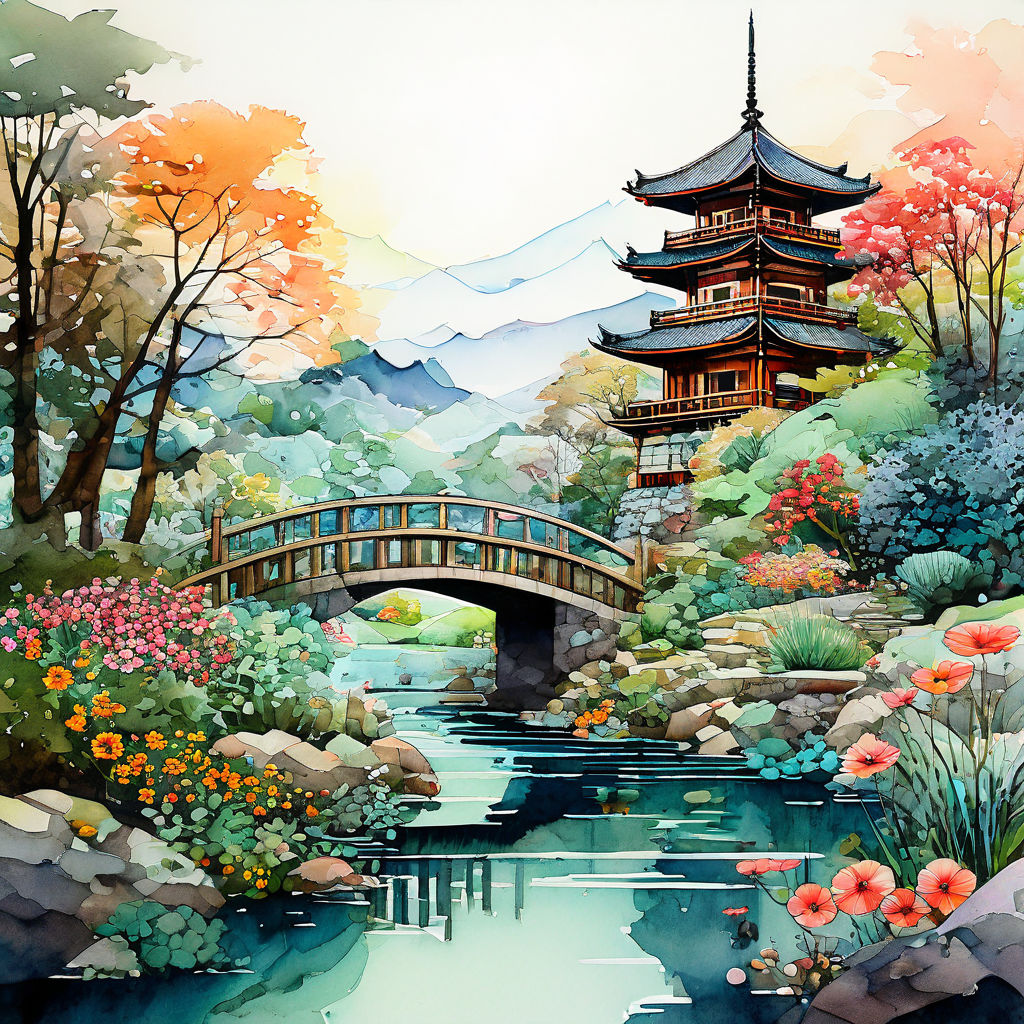The image depicts a bright and cheerful Japanese garden scene captured in a highly detailed, animated drawing. Dominating the right side of the picture is a brown, wooden pagoda building with three floors, each topped with distinct black roofs extending outwards. At the apex of the structure, a spear-like ornament reaches skyward. The pagoda is set atop a stone foundation, adding to its impressive stature. Surrounding the building is a colorful garden in full bloom, indicating the vibrancy of spring. 

The garden is filled with an array of flowers in hues of orange, red, peach, and pink, scattered among the bright green trees and bushes that frame both sides of the scene. In the very center of the image, a gently flowing blue stream bisects the garden, spanned by a slightly rounded, gray and beige bridge. The bridge acts as a connective element, linking the left and right sides of the garden. Rocks and patches of grass lie along the stream's edges, adding natural texture to the scene.

Above, the sky appears brightly lit and white, possibly due to natural lighting, and is complemented by distant mountains that softly backdrop the composition. The overall setting exudes clarity and a sense of serene natural beauty.